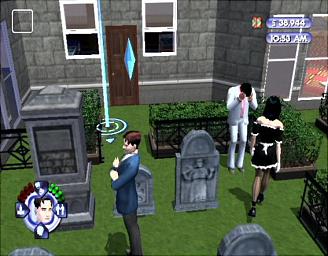A detailed descriptive caption for the given image could be:

"The scene appears to be a screenshot from a video game, likely The Sims. It depicts a somber setting in a graveyard. In the background, a gray house with two visible windows and a brown door partially frames the scene. Prominent in the foreground is a large monument along with several smaller gray headstones. On the left side, a man dressed in a blue suit stands facing left, marked by a blue diamond hovering above his head, indicating he is an active Sim. Behind him, a French maid can be seen walking. In the center foreground, another man with black hair, dressed in a white suit, is crouched down with his head in his hands, suggesting a moment of grief or despair. The timestamp on the image reads 10:33 a.m., hinting at the time of the in-game event."